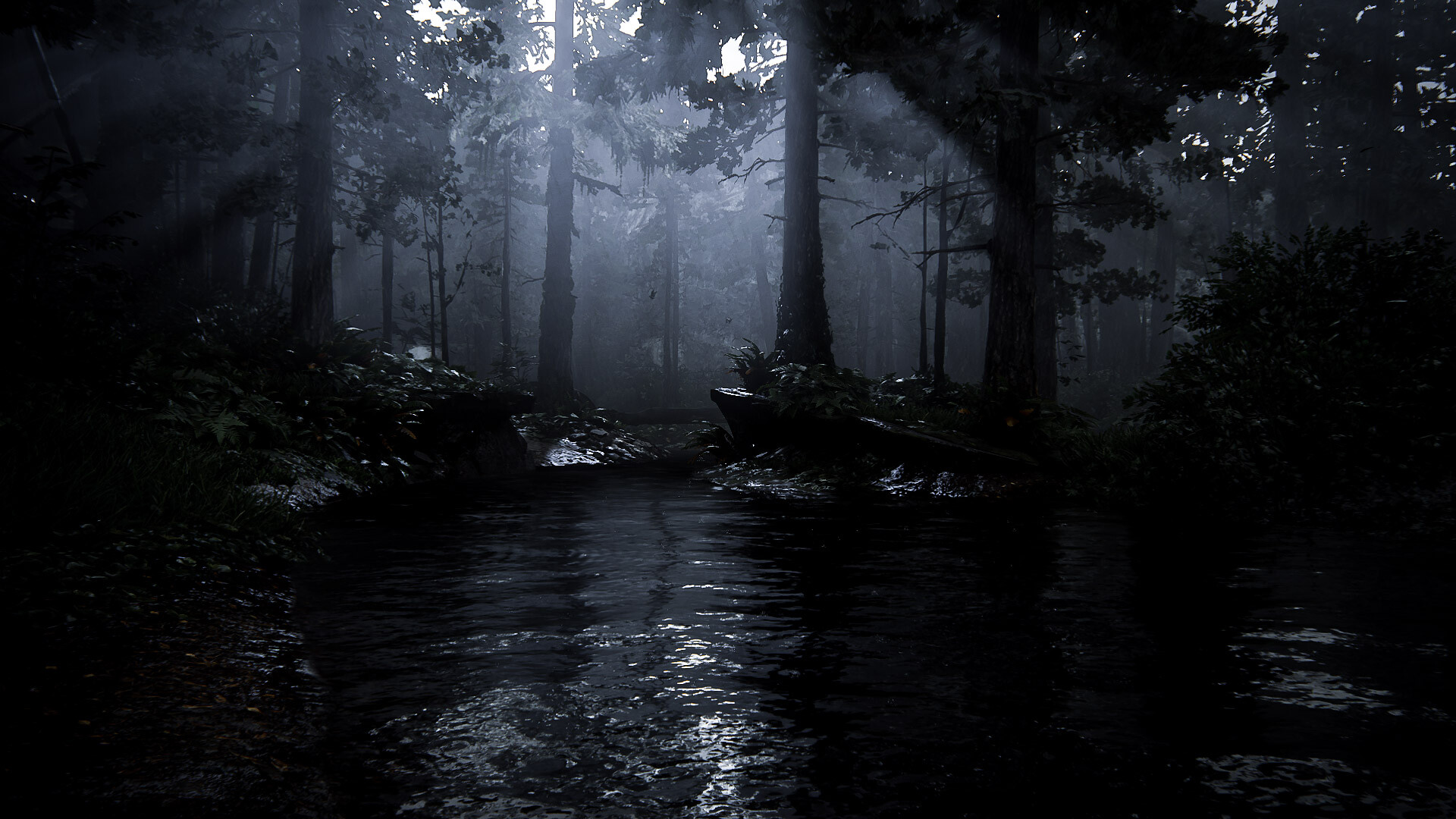The image depicts a serene pond surrounded by dense forest, captured during twilight. Though it’s dark, the sky above emits a subtle glow that gently illuminates the scene, allowing visibility of the immediate surroundings. The pond itself has a wet, rocky edge with the sky’s light beautifully reflecting off its surface. Towering trees, predominantly pine interspersed with a few deciduous ones, envelop the area so densely that it’s impossible to see beyond them. The forest creates a thick, impenetrable barrier of foliage. The left and right edges of the image are especially shrouded in darkness, with the dwindling light failing to penetrate these areas, adding a sense of depth and mystery to the tranquil landscape.